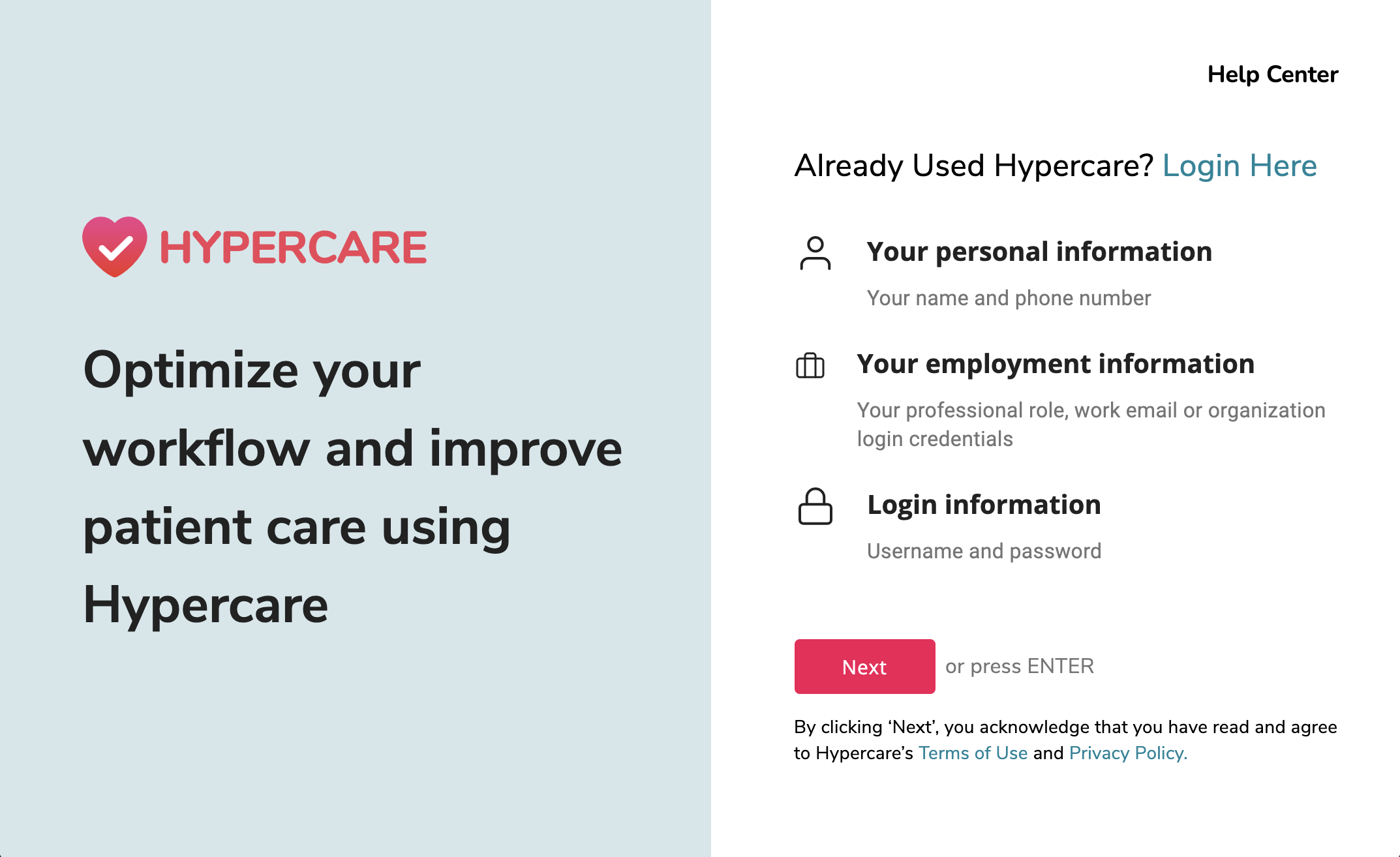The HyperCare page is visually divided into two distinct halves. On the left, a gray background showcases a heart icon with a white checkmark inside it, symbolizing care and approval. Beside the icon, in bold red uppercase letters, is the word "HYPERCARE." Following this, bold text reads, "Optimize your workflow and improve patient care using HyperCare."

The right side features a white background. At the top right corner, the text "Help Center" is displayed. Below, the text reads, "Already used HyperCare? Log in here," with "log in here" highlighted in blue. Further down, there is an icon of a person accompanied by the text "Your personal information," specifying "Your name and phone number." Next is an icon of a briefcase, with the label "Your employment information" followed by "Your professional role, work email, or organization login credentials." Beneath this, a padlock icon appears with the words "Login information," detailing "Username and password." At the bottom, a centrally placed red rectangular button contains the word "NEXT" in white text. Below this button, in capital letters, is the instruction "OR PRESS ENTER." A note specifies that by clicking "NEXT," users acknowledge they have read and agreed to HyperCare's "terms of use" and "privacy policy," with both terms highlighted in blue.

The clean, structured design of the page guides users through the login process with clarity, ensuring they are informed about the terms and privacy policy.